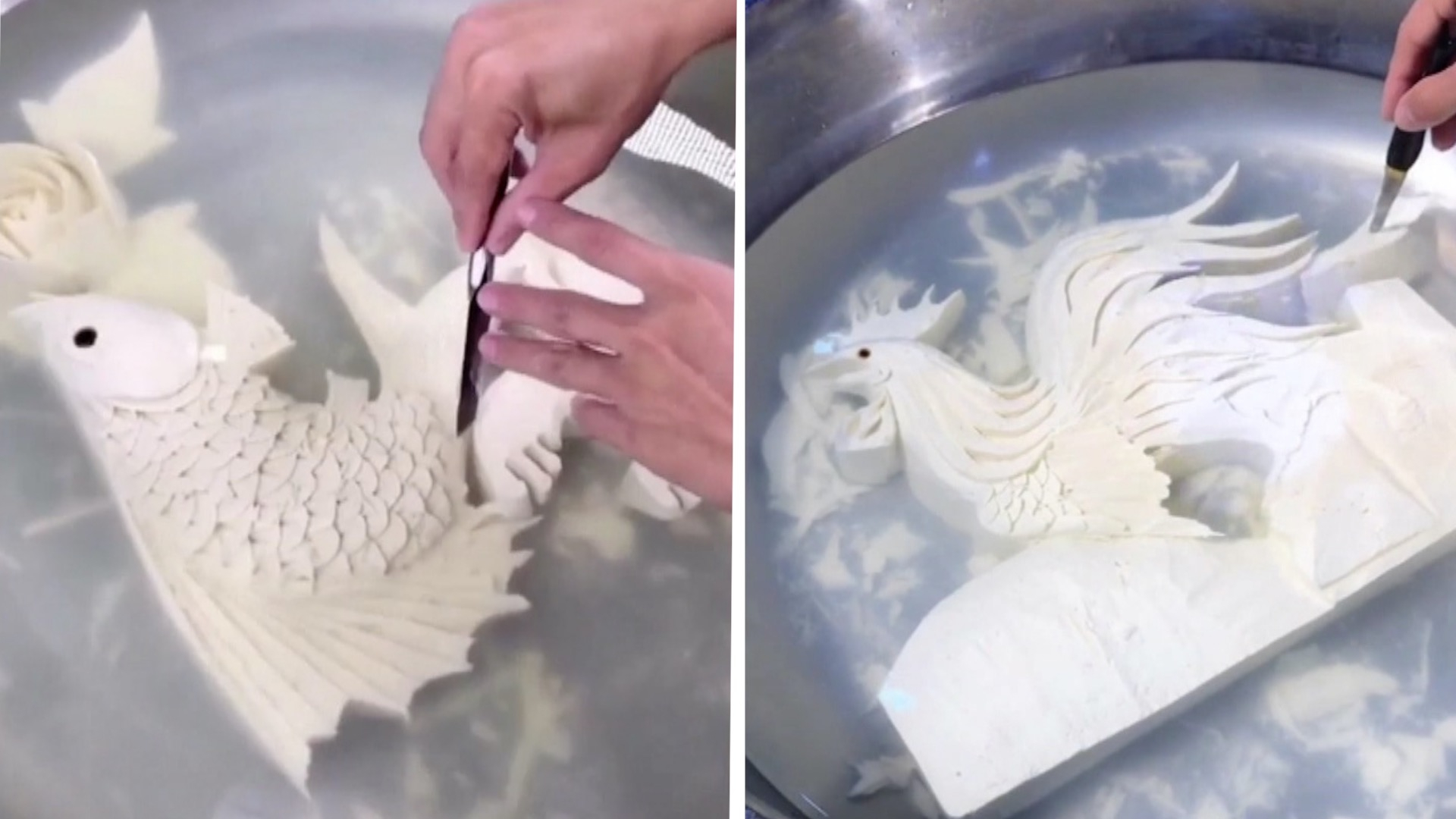This is a color side-by-side photograph capturing the meticulous process of a man carving intricate designs into a white plaster-like material, submerged in a large stainless steel bowl filled with a milky water solution. On the left image, the carver's lighter-skinned hands, emerging from the right corner of the frame, delicately hold a razor-like carving knife with his left hand, skillfully shaping a koi fish. The fish features highly detailed scales and a distinct black circular eye, with its body oriented sideways and facing upwards. The water surrounding the koi is a transparent milky white, adding to the serene ambiance of the scene. Moving to the right image, the focus shifts to the man's hand in the top right corner, holding the same razor-like knife as he carves the form of a rooster. The rooster, lying in the same milky solution, displays finely crafted long feathers and yet another black circular eye, with remnants of plaster sinking to the bottom of the bowl, illustrating the extent of the detailed craftsmanship involved.